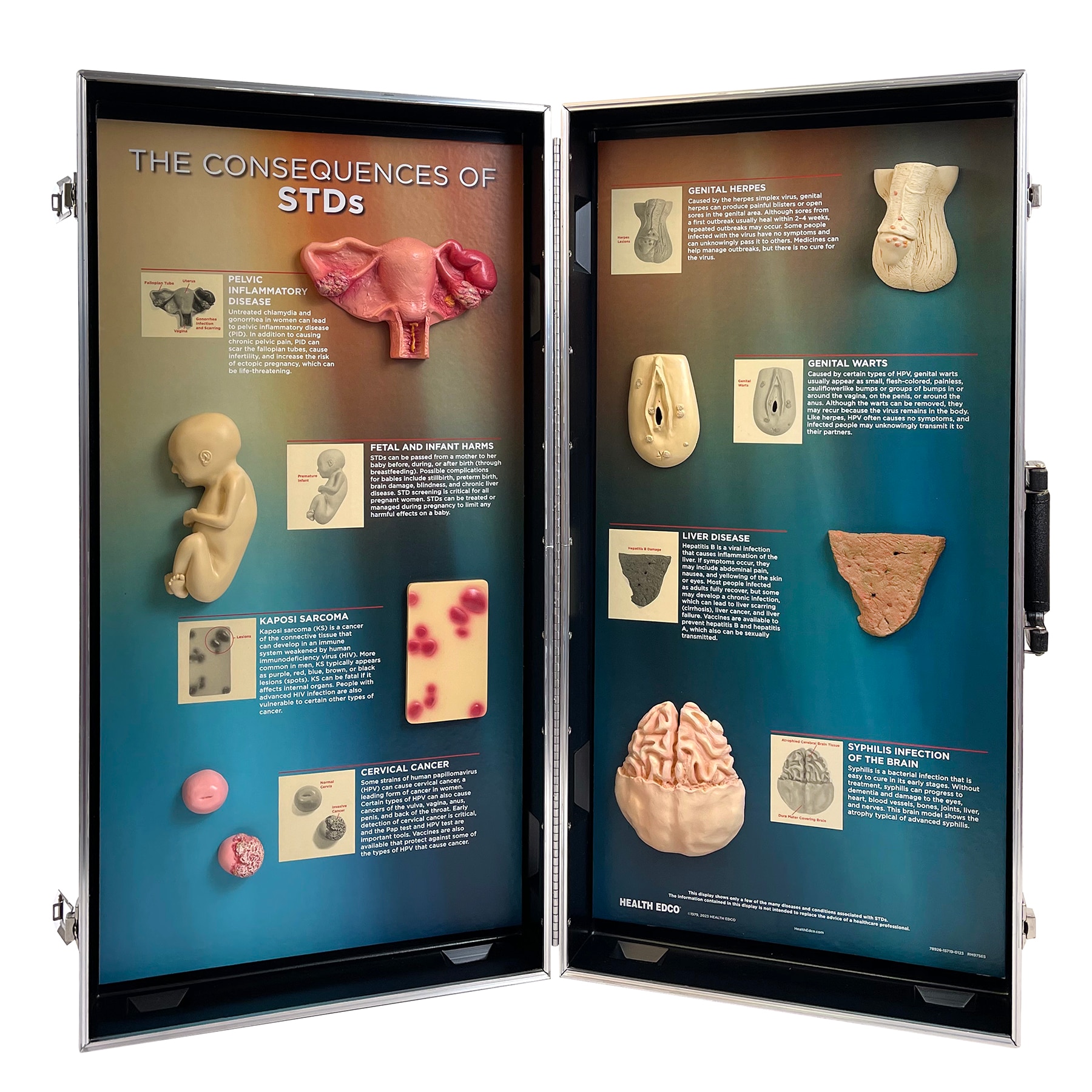This detailed display, designed for educational settings such as fairs, career fairs, or conferences, is a hinged, two-sided board that locks on each side and features a black handle on the right. The background showcases a gradient of continuous rainbow colors, transitioning from yellow and red at the top to blue at the bottom. The top left section of the display prominently features the title "The Consequences of STDs," written in white capital letters with black borders. The left side displays various health impacts with detailed 3D models: a pink pelvis illustrating pelvic inflammatory disease, a white baby representing fetal and infant harms, red bumps against a yellow background for Kaposi's sarcoma, and textured pink circles for cervical cancer. The right side includes more 3D models: a white penis with bumps indicating genital herpes, a white vagina with similar growths for genital warts, a brown, textured liver to represent liver disease, and a pink brain model labeled as a syphilis infection of the brain. In the bottom left-hand corner, the display is branded with "health EDCO."